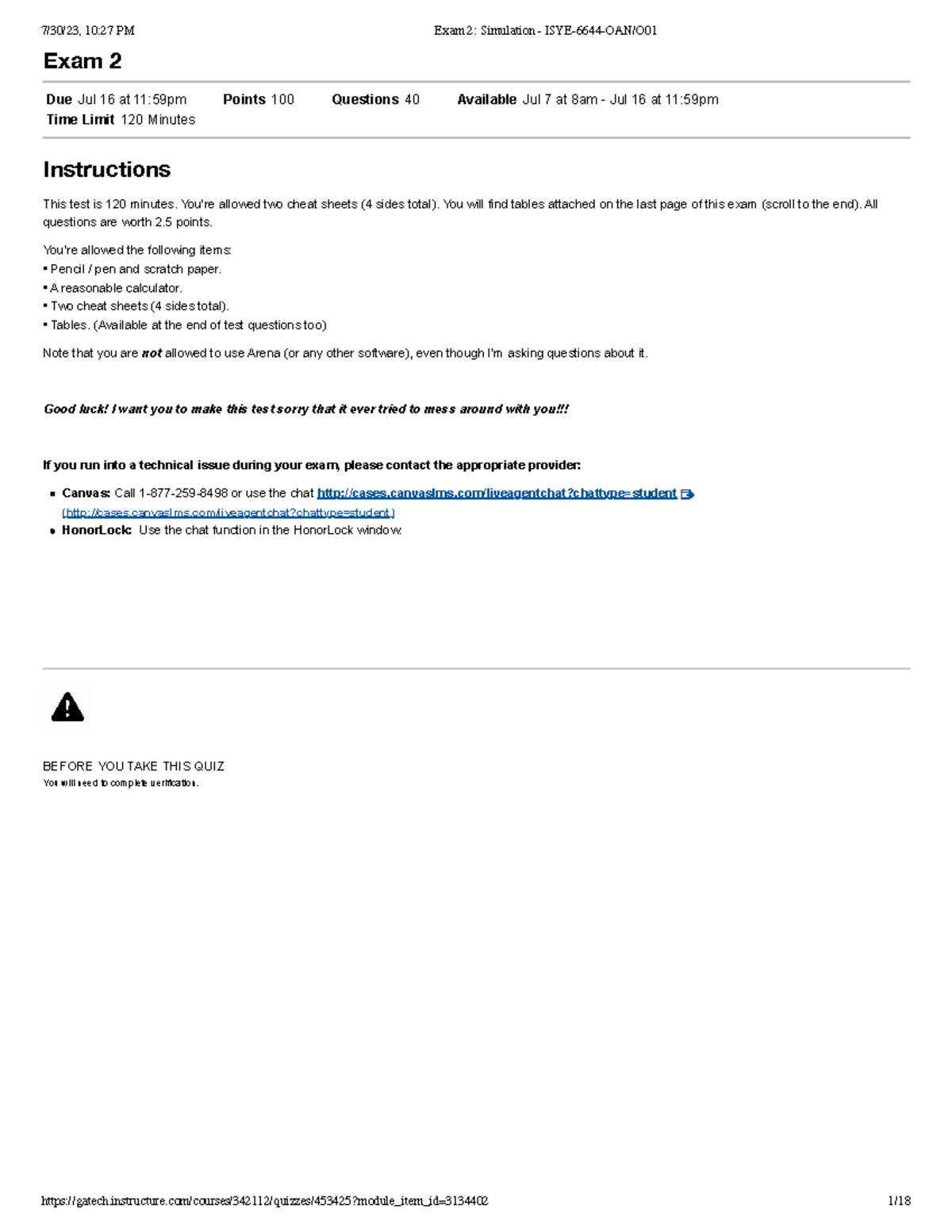In the screenshot, the top left corner displays the date "7/30/23 10:27 p.m." To the immediate right, text reads: "Exam 2 Simulation" followed by what appears to be a course code or identifier "YE 666440 AN 001". Below, the due date for Exam 2 is indicated as "July 16th at 11:59 p.m." with a total of 100 points available for 40 questions. The exam can be accessed starting from "July 7th at 8:00 a.m." until "July 16th at 11:59 p.m."

The instructions are written in bold black text, stating: "This test is 120 minutes. You are allowed two cheat sheets (four sides total). You will find tables attached on the last page of this exam; scroll to the end. All questions are worth 2.5 points each. You are allowed the following items: pencil or pen, scratch paper, a reasonable calculator, and two cheat sheets (four sides total). Additionally, reference tables are provided at the end of the exam."